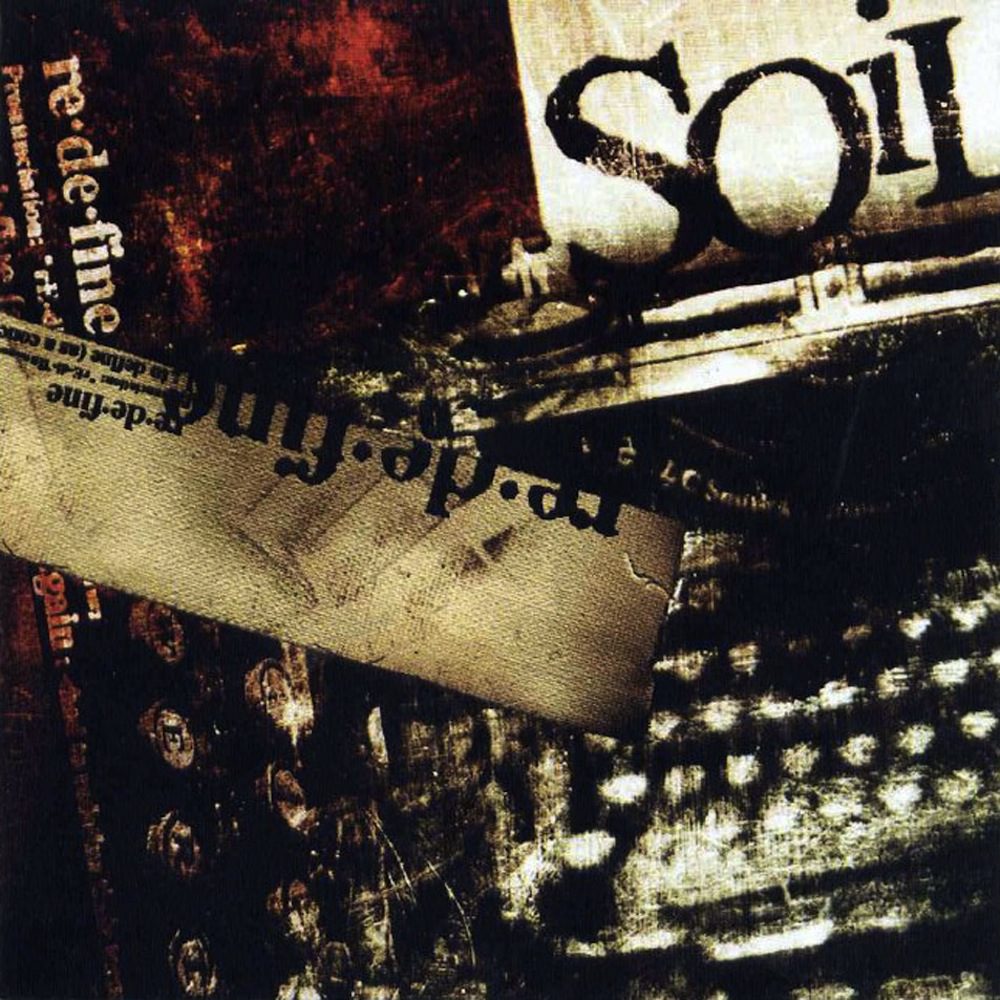This photograph features a dark and intriguing collage that primarily uses black, white, and red colors. Dominating the image are two distinct sections of text. On the upper part, the word "Soil" is prominently displayed in large, bold, black print, styled in an aerial typewriter font, suggesting a vintage aesthetic. Directly beneath, a canvas-stained strap crosses the middle of the image, adding texture and depth. Below the strap, we see the title "Re.D.e.F.i.n.e," which seems to be the name of a musical release by the band Soil, typed in the same vintage typewriter font, though partly upside down, enhancing the artistic disarray. In the bottom-left corner, some typewriter keys are visible, giving off the impression of an old typewriter, further emphasizing the retro theme of the photograph. No people are present, and there is no date, location, or other identifying information. In certain areas, the text appears blurry, making it difficult to read. The entire composition measures approximately five by five.